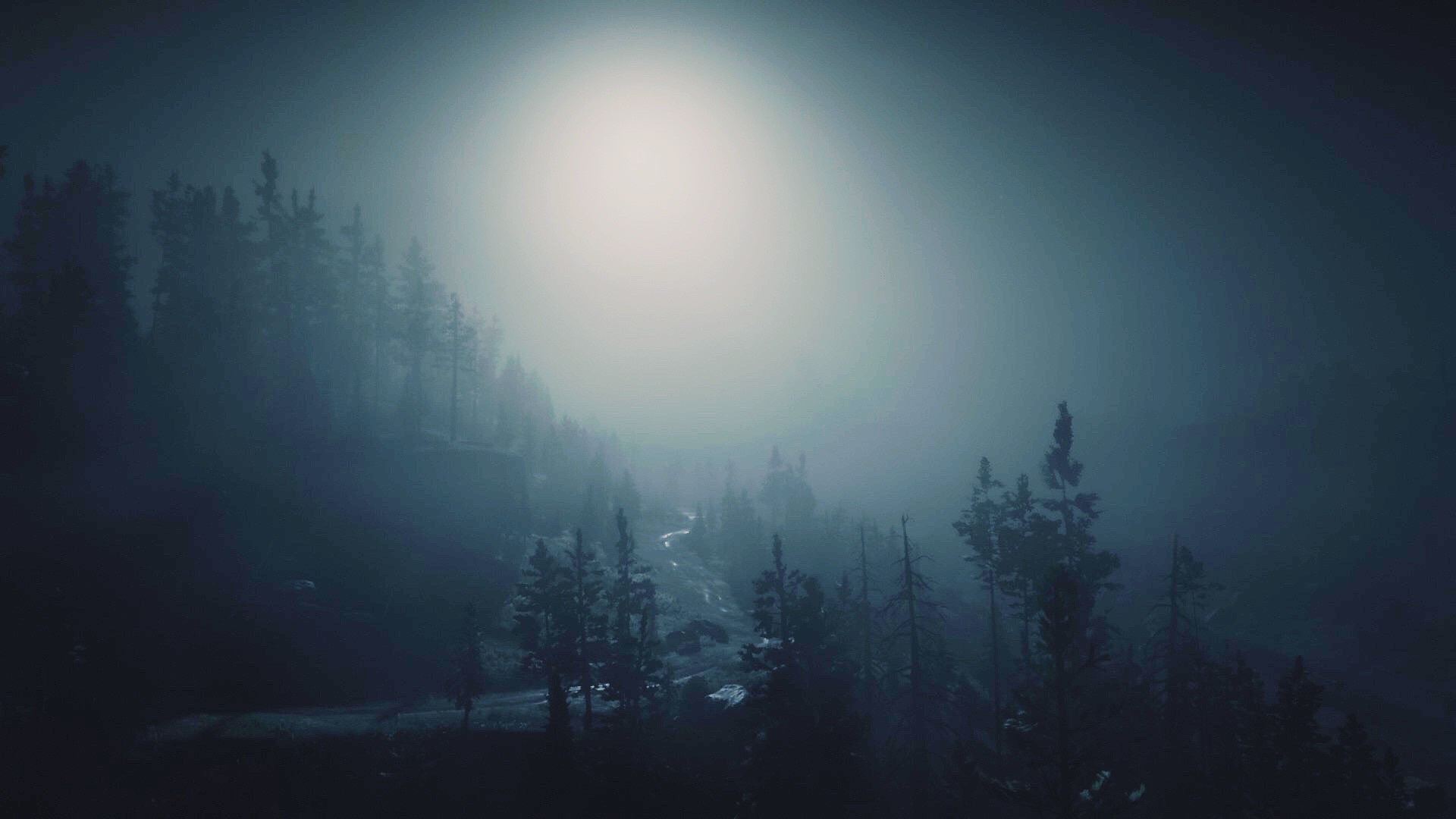The image captures a serene and secluded woodland scene at night. Dominating the center of the picture is an exceptionally bright light, likely the moon, casting an ethereal glow over the landscape. Tall trees crowd the top left and bottom right corners of the image, their imposing silhouettes stark against the illuminated background. A narrow dirt road winds its way from the bottom left corner, through the center, and up towards the radiant sky, inviting the viewer to ponder where it might lead. The sky itself is strangely bright, creating a surreal atmosphere, except for the top left and right edges, which remain cloaked in darkness. No signs of human presence or activity can be seen, adding to the sense of tranquility and isolation.